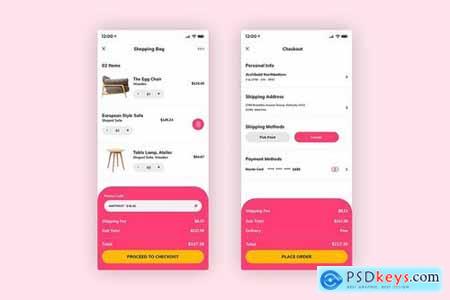This image appears to be a stock photo used for an advertisement, likely related to an e-commerce platform like Klarna. It features two smartphones displayed side by side against a pink background, reminiscent of Klarna's branding. Each phone screen shows different product listings; the left phone screen displays a chair resembling an Ikea design alongside a small four-legged stool. The right phone screen seems to prompt the user to provide details or proceed with a purchase, suggesting functionalities typical of an online shopping interface. The presence of the website URL "PSDKeys.com" adds a layer of ambiguity, which might indicate the image is sourced or edited from there. Overall, the image could be part of a tutorial or advertisement showing how to shop for furniture items through Klarna's platform.